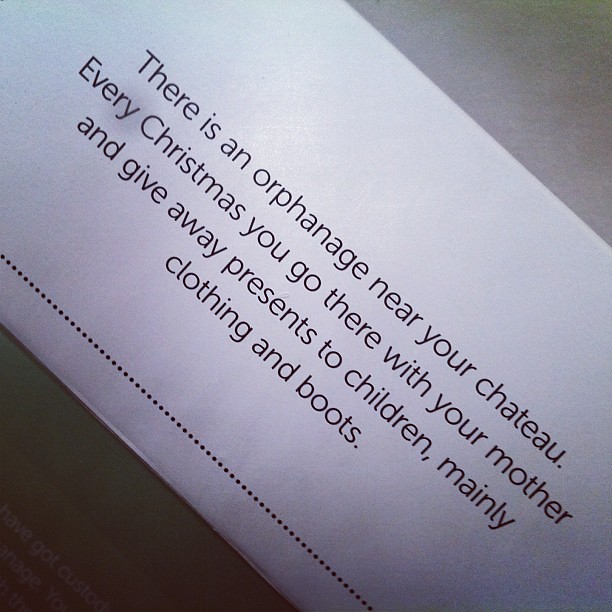The image depicts a worn piece of white paper placed on a gray table, photographed at an angle, making the text run diagonally from the top left to the bottom right. The message, written in black ink, reads: "There is an orphanage near your chateau. Every Christmas you go there with your mother and give away presents to children, mainly clothing and boots." The paper bears visible shadows and faint dinginess, with a notable presence of dotted lines at the bottom of the message. In the upper left corner and lower right corner of the photo, a brown background is faintly visible, and there is a suggestion of some additional faint text near the bottom left. The entire scene is illuminated, casting mild shadows and highlighting areas of the paper, potentially adding a slight red tinge in the lower part of the text.